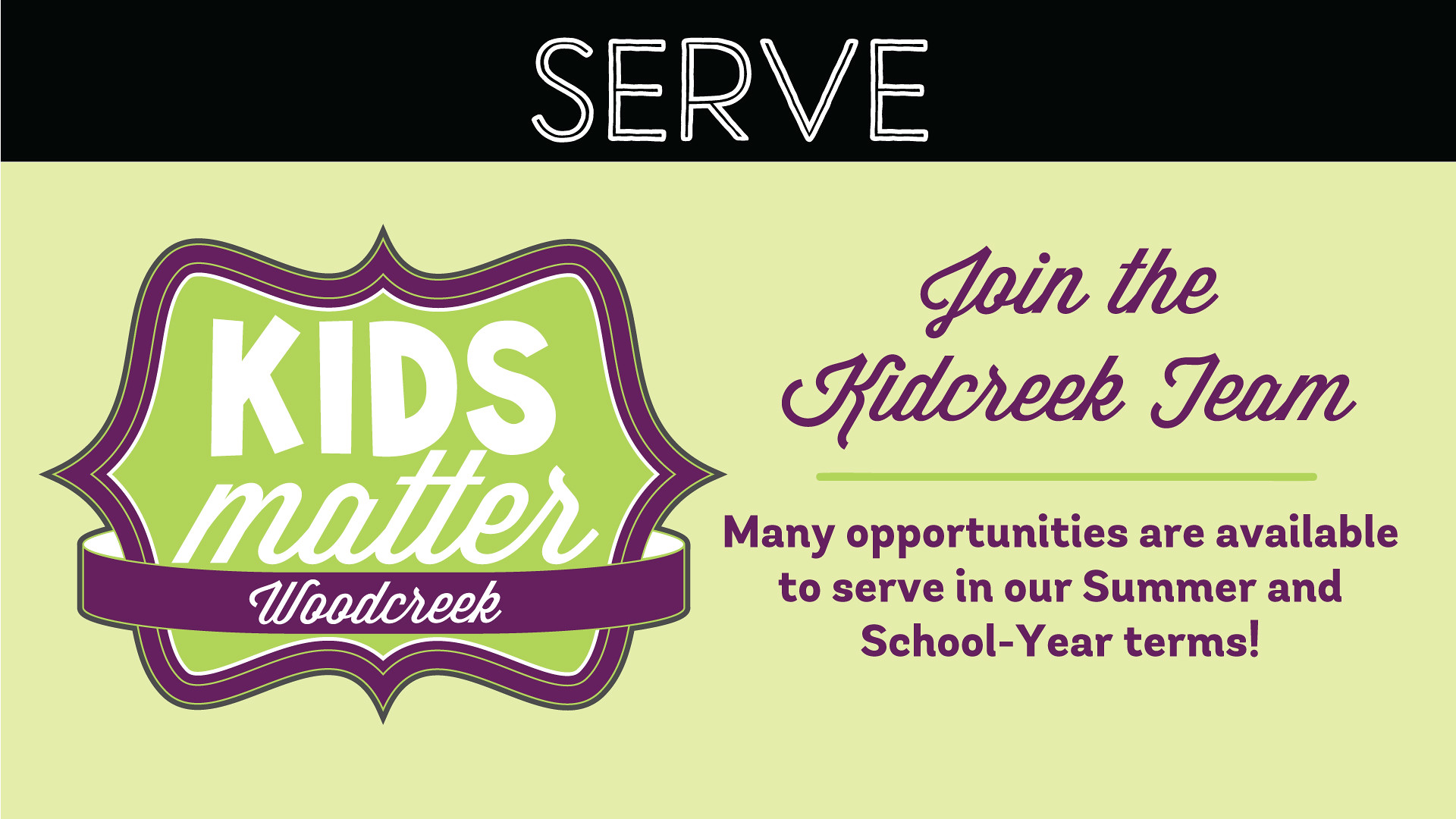This rectangular online ad features a striking design with a unified message. At the top, a black horizontal bar displays the word "SERVE" in bold, all-caps white letters. The main background of the ad is a soothing mint green. On the left side, a prominent logo is crafted like a badge, outlined in purple with a bright green interior. This badge contains the text "Kids Matter" in white, and it's accented by a purple banner with the words "Wood Creek" in white cursive. To the right of the badge, in elegant purple cursive, the ad invites viewers to "Join the Kid Creek Team." Below this, separated by a green line, additional text in purple states, "Many opportunities are available to serve in our summer and school year terms." Overall, the ad combines engaging colors and fonts to effectively communicate its call to action.